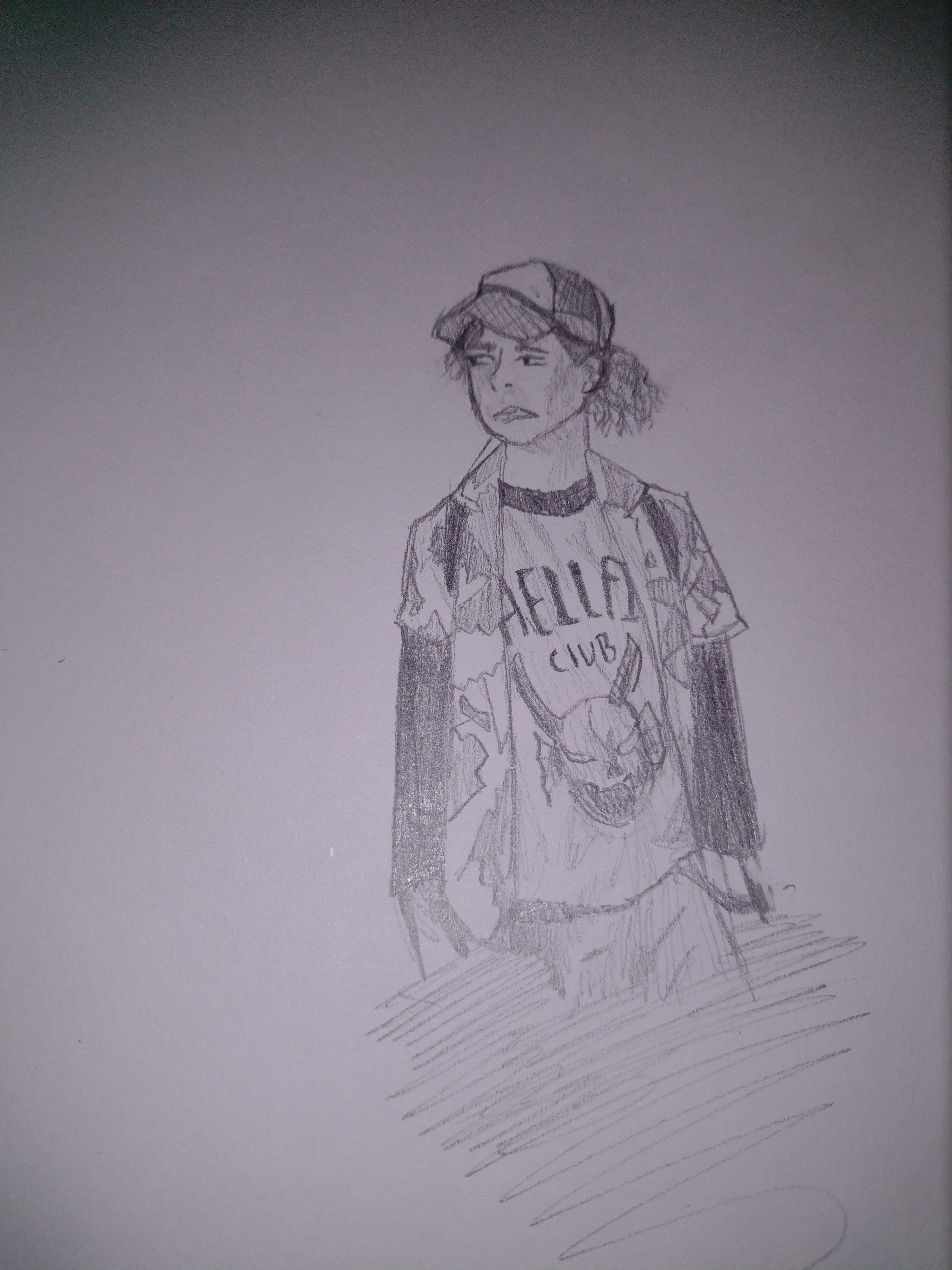The image is a darker photograph of a pencil sketch on plain white paper, capturing a detailed rendering of a character with longish, wavy hair that doesn't quite reach their shoulders. The person is wearing a baseball cap with the bill obscuring their face slightly, casting a shadow over eyes that gaze pensively to the left, conveying a sense of worry. The facial expression is tense, with a mouth turned down in apprehension. 

The character is dressed in a layered outfit: a short sleeve, camouflage-type jacket or overshirt on top of a long sleeve dark baseball shirt. The baseball shirt has a dark collar and features the words "Hellfire Club" along with an image of a devilish figure with horns. The hands and legs of the figure are less defined, fading into scribble lines at the bottom of the sketch. The sketch carries an amateurish, fan-drawn quality, possibly depicting Eddie Munson from the show Stranger Things. The overall image has dark, shadowy edges with varying shades of gray, contributing to its unfinished, raw appearance. Detailed pencil strokes suggest the presence of a backpack, with dark gray lines indicating straps over the shoulders, completing the thoughtful composition.